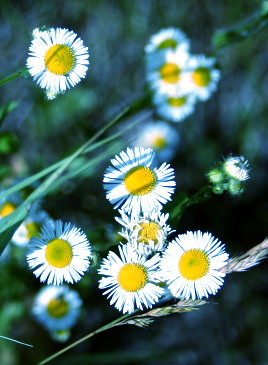This vertical, rectangular photograph captures a close-up of approximately 10 to 12 daisies in full bloom. These flowers, characterized by vibrant yellow centers comprised of numerous small yellow pieces, resemble rounded button-like structures. Encircling these centers are numerous dainty, white petals – each flower boasting between 50 to 100 of these delicate, bright white petals. The daisies are attached to green stems that flow diagonally across the frame, some angling downward. The background is a blend of blurred daisies and thick vegetation with a bluish-green tint, suggesting a woodsy setting. The overall hue of the image has a subtle blue tone, adding a serene and slightly cool atmosphere to the vibrant floral scene.